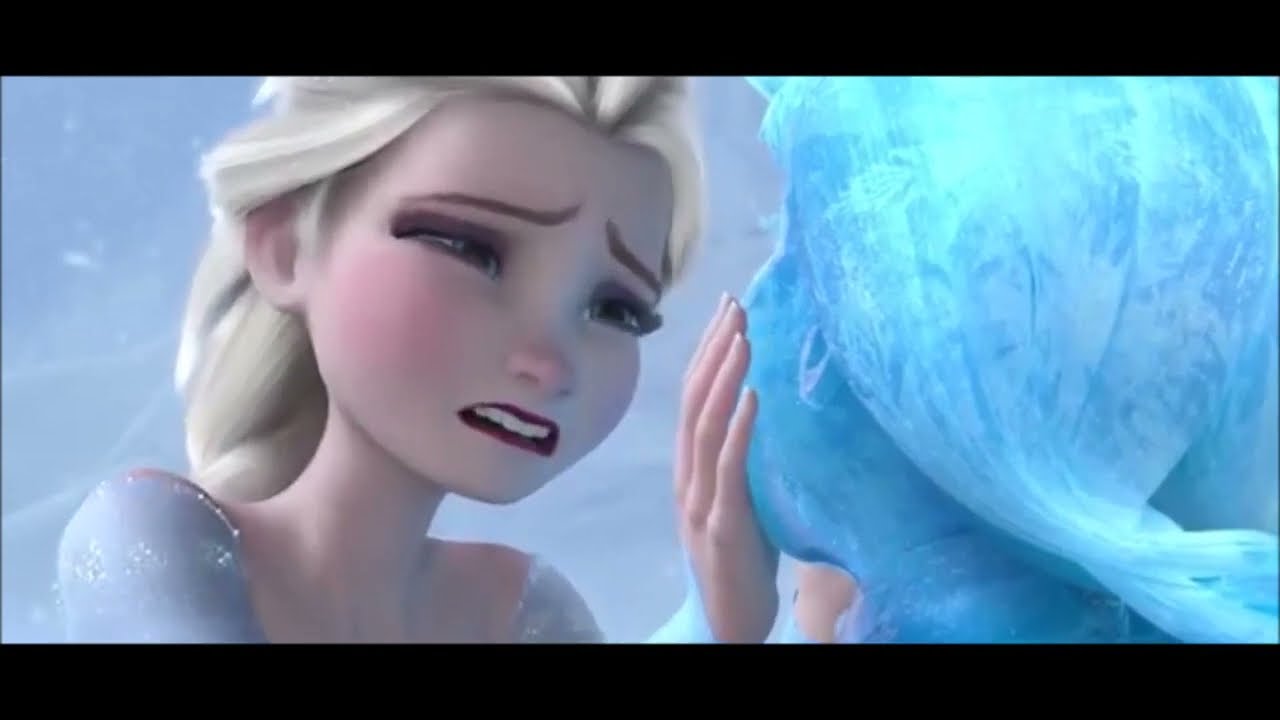This is a detailed still shot from Disney's animated movie Frozen. The image captures a close-up, shoulder-up view of Elsa, positioned on the left side of the landscape-oriented frame. Elsa is depicted in distress, with a sad, anguished expression on her face, red lipstick, and a silvery gown, her hand tenderly touching the cheek of a character on the right side who appears frozen and is rendered in icy blue hues. The frozen figure is seen from behind. The image's color palette includes various shades of blue, light blue, aqua blue, black, white, gray, Elisabeth's blonde hair, dark red lipstick, and some beige. The setting is a poignant, emotionally charged moment typical of the animated style in Disney's Frozen.